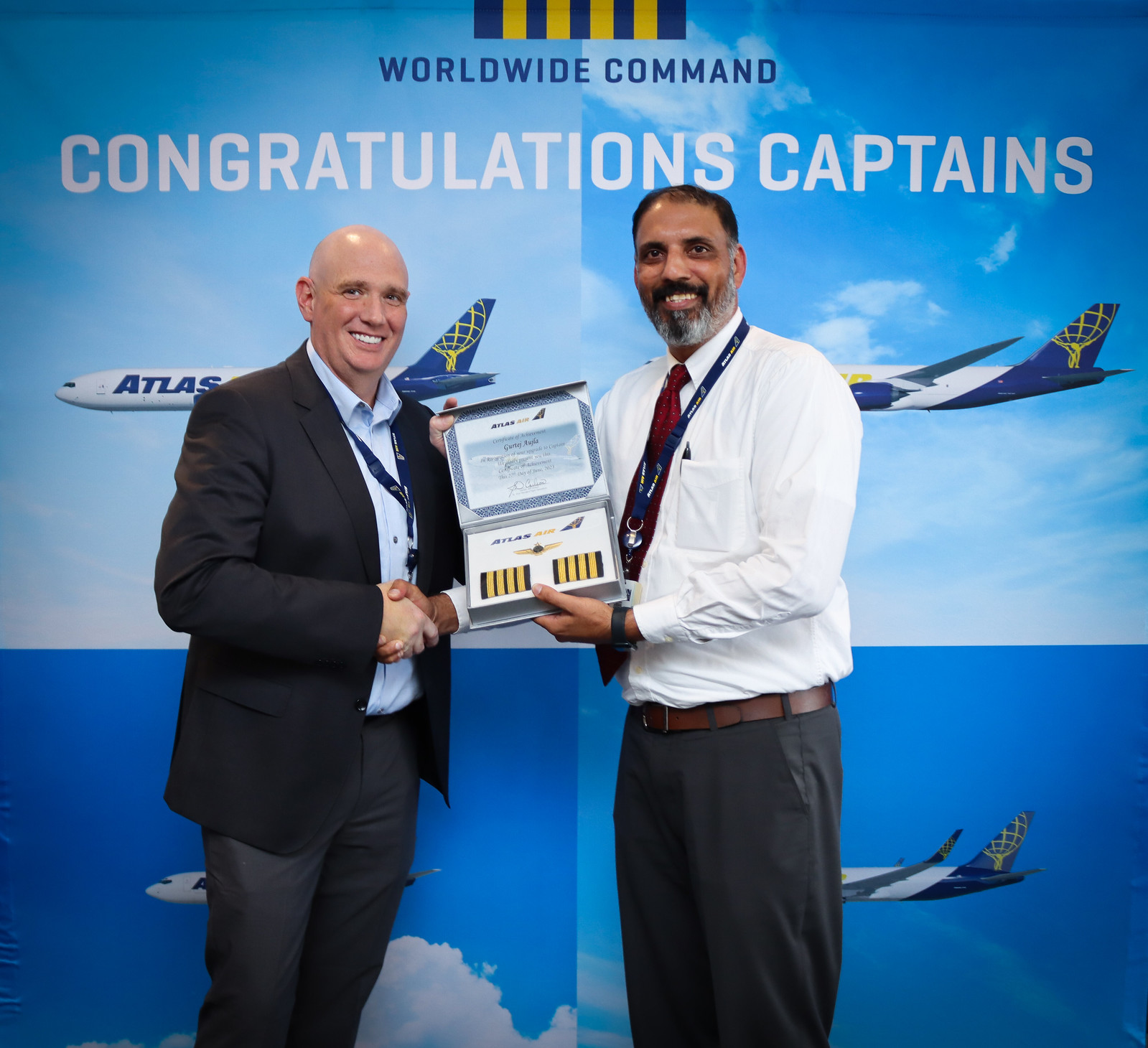In this photograph of an award ceremony, two men, who appear to be in their 50s, are shaking hands and smiling at the camera, standing in front of a large banner that dominates the background. The banner features four photographs of jet planes in mid-flight against a backdrop of blue skies and clouds, with "Worldwide Command" inscribed at the top followed by "Congratulations Captains." The man on the left, who is bald and has a light complexion, is dressed in a dark suit jacket with a light blue button-up shirt and black pants. The man on the right, who has a darker complexion and a gray beard, is slightly taller and balding. He is wearing a white collared shirt with a red tie, a blue lanyard, and dark slacks. Between them, they are holding an open box that contains a certificate and pilot epaulettes, possibly indicating the conferment of captain's stripes and wings. The celebratory moment captures the essence of achievement and camaraderie in the aviation field, with both men embodying pride and accomplishment.